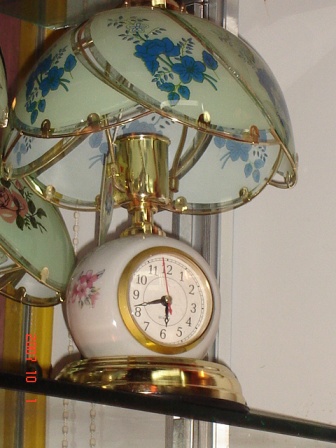The photograph captures a unique combination of a clock and lamp with an ornate, vintage styling, reminiscent of early 1900s Tiffany designs. The base is a round, gold structure adorned with a white ceramic section that features a traditional clock. The clock face is white with black hour and minute hands, and a red second hand currently almost at the 12, with black numerals from 1 through 12. The ceramic portion also displays a delicate pink flower. 

The lamp extends above this clock, featuring a glass shade with a white floral background and blue floral patterns. The inner structure of the lamp is bright gold, with the lampshade shaped like teardrop petals outlined in golden brushed steel. The shade also includes an olive-colored glass with blue petal details and dark green leaves. The cylindrical centerpiece where the light bulb fits resembles a chalice. 

There is a red timestamp on the clock reading "2007-10-1," and the backdrop features a white wall with a silver-colored metal strip, possibly part of a door frame. Additionally, another smaller lamp with a similar design, but with pink and white petals, is partially visible in the frame, hinting at a collection or a matched set.